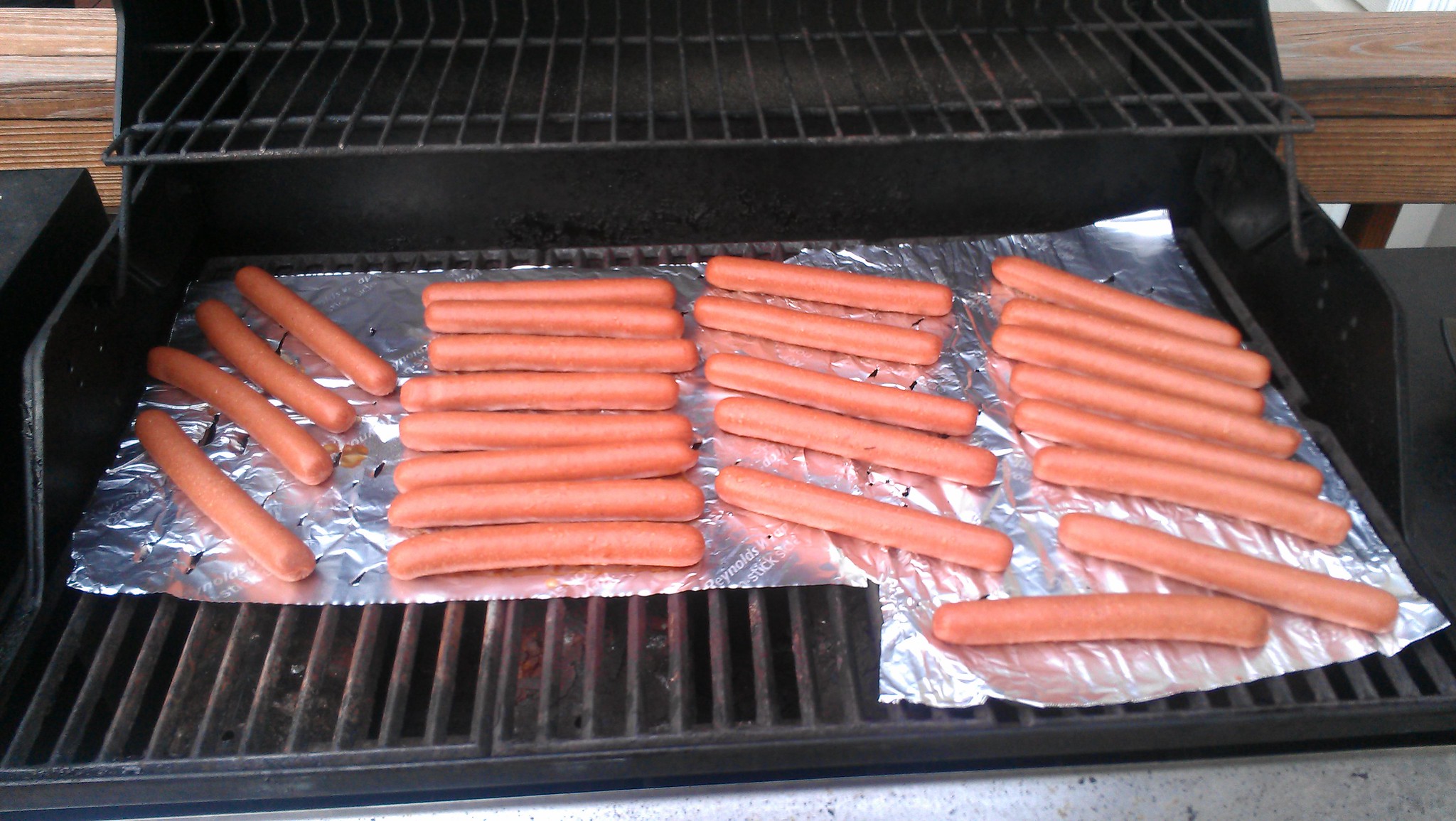In the image, we see a well-used outdoor grill set against a backdrop of light reddish-brown wood panels that run horizontally. The grill itself has dark gray and black components, including a hood at the top and a series of three dark gray racks at the bottom, with an additional rack sitting above for warming. The primary rack is covered with aluminum foil, arranged in two overlapping pieces—one horizontal and one vertical to the right. On the foil, there are multiple columns of uncooked hot dogs, totaling over a dozen. The first column has four hot dogs arranged diagonally, the second column has eight hot dogs packed tightly in a horizontal line, the third column features five hot dogs arranged vertically, and the fourth column has another eight hot dogs loosely tilted vertically. Behind the grill, the wooden deck railing is visible, adding to the outdoor setting of the scene.